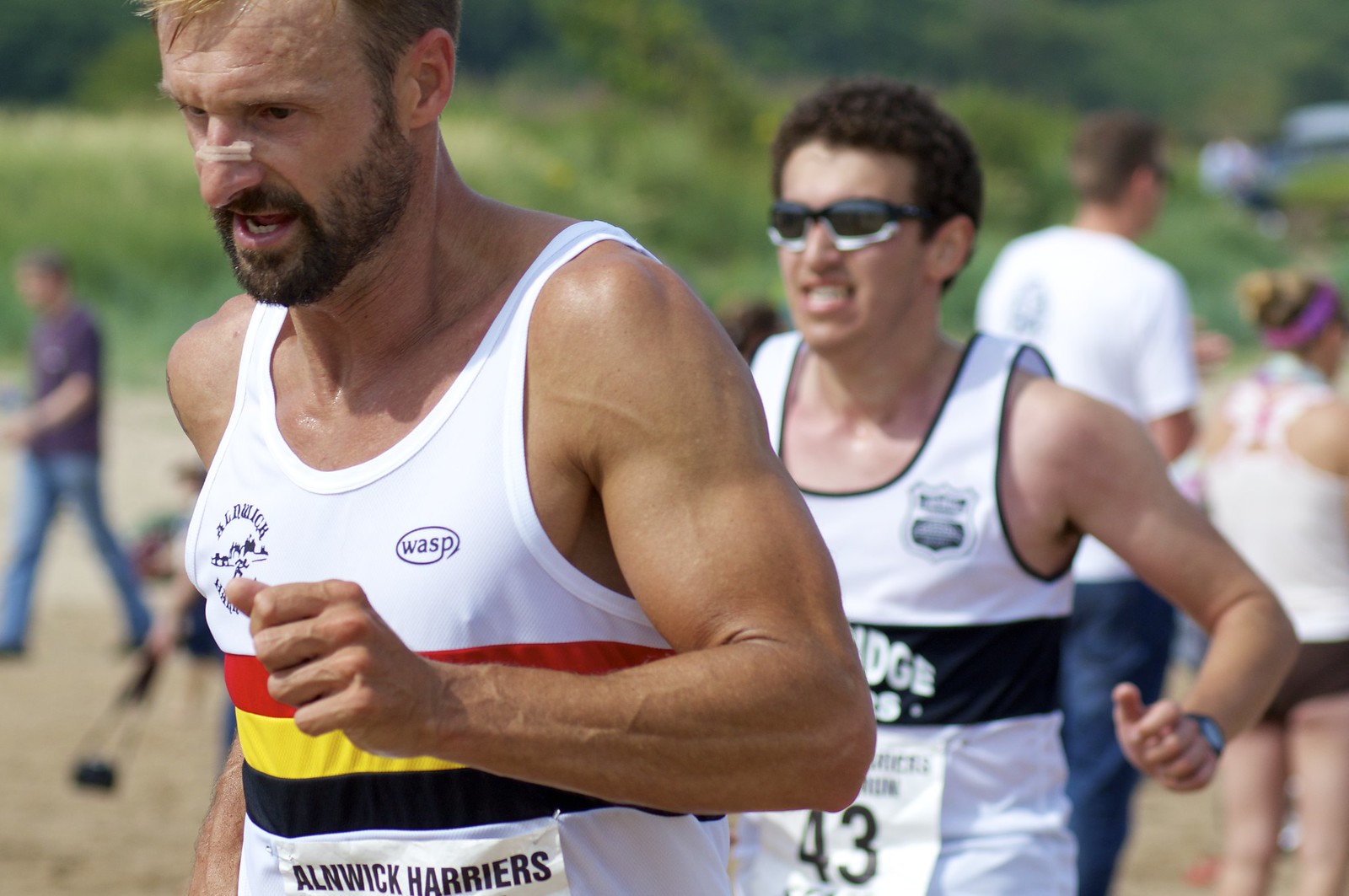In this full-color outdoor photograph bathed in nice weather, two Caucasian men are captured running in what appears to be a race. The man in the foreground, who sports a light beard and a nasal strip for breathing, is clad in a white tank top emblazoned with red, yellow, and black, likely symbolizing the German flag. His race bib, displaying the name "Alnwick Harriers," is partially obscured, making the number unreadable. He appears fit and determined. Trailing him is another man, adorned with running sunglasses and wearing a similar white tank top featuring a black stripe around the torso. His race bib clearly shows the number 43. In the background, there are several onlookers facing away from the race, engaged in their own activities. These include a woman in shorts, a man in a white t-shirt, and another individual on the far left in a blue-purple t-shirt, who seems to be walking in the general direction of the runners but not focusing on the race.